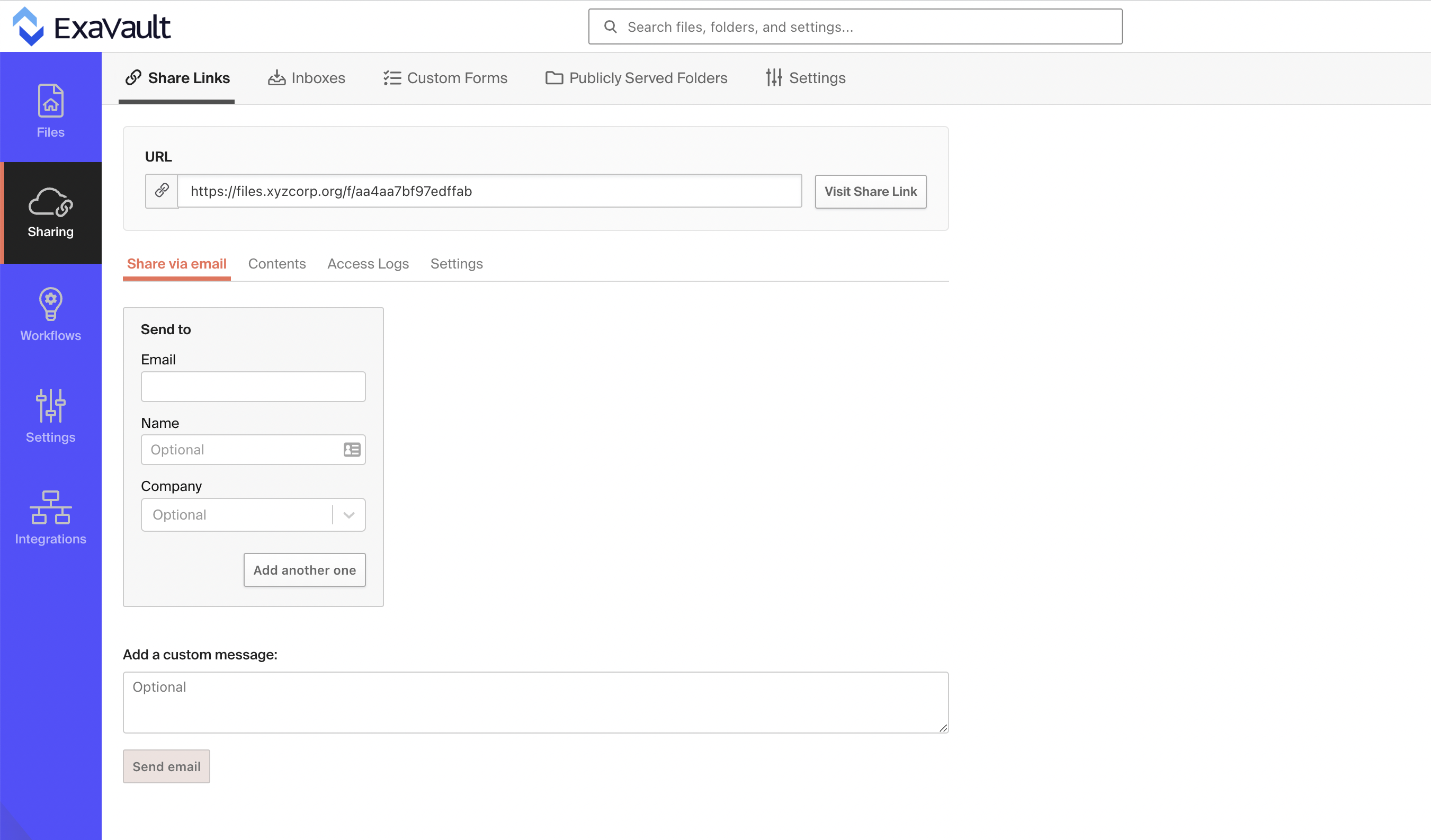The image features a user interface with a white background. At the top, the word "EXAFOT" is prominently displayed, accompanied by a pair of arrows—one blue pointing up and one dark blue pointing down—that indicate navigation options. Below this, a search bar is centrally positioned with the placeholder text "Search files, folders, and settings."

On the left side, there is a vertical navigation menu with several sections, each represented by an icon: 
- **Files**
- **Sharing** (highlighted in black, indicating it is selected)
- **Workflow**
- **Settings**
- **Integrations**

The main content of the page is structured around several sections. At the top, there’s a horizontal navigation bar featuring:
- **Share Links** (underlined in black, indicating it is selected)
- **Inboxes**
- **Custom Forms**
- **Publicly Served Folders**
- **Settings**

Directly below this bar is a gray URL input box containing the URL "https://files.xycorp.org," followed by a "Visit Share Link" button on the right. 

Below the URL box, another horizontal navigation bar, marked with sections such as:
- **Share via Email** (underlined in red, indicating it is selected)
- **Contents**
- **Access Log**
- **Settings**

The "Share via Email" section includes several input fields:
- **Send To**: A gray box labeled "email" (currently blank), with optional fields for "Name" and "Company" also left blank.
- An "Add Another One" button to add additional recipients.
- An "Add a Custom Message" entry box, labeled as optional, which is also blank.

Finally, at the bottom of this section, there is a prominent "Send Email" button.